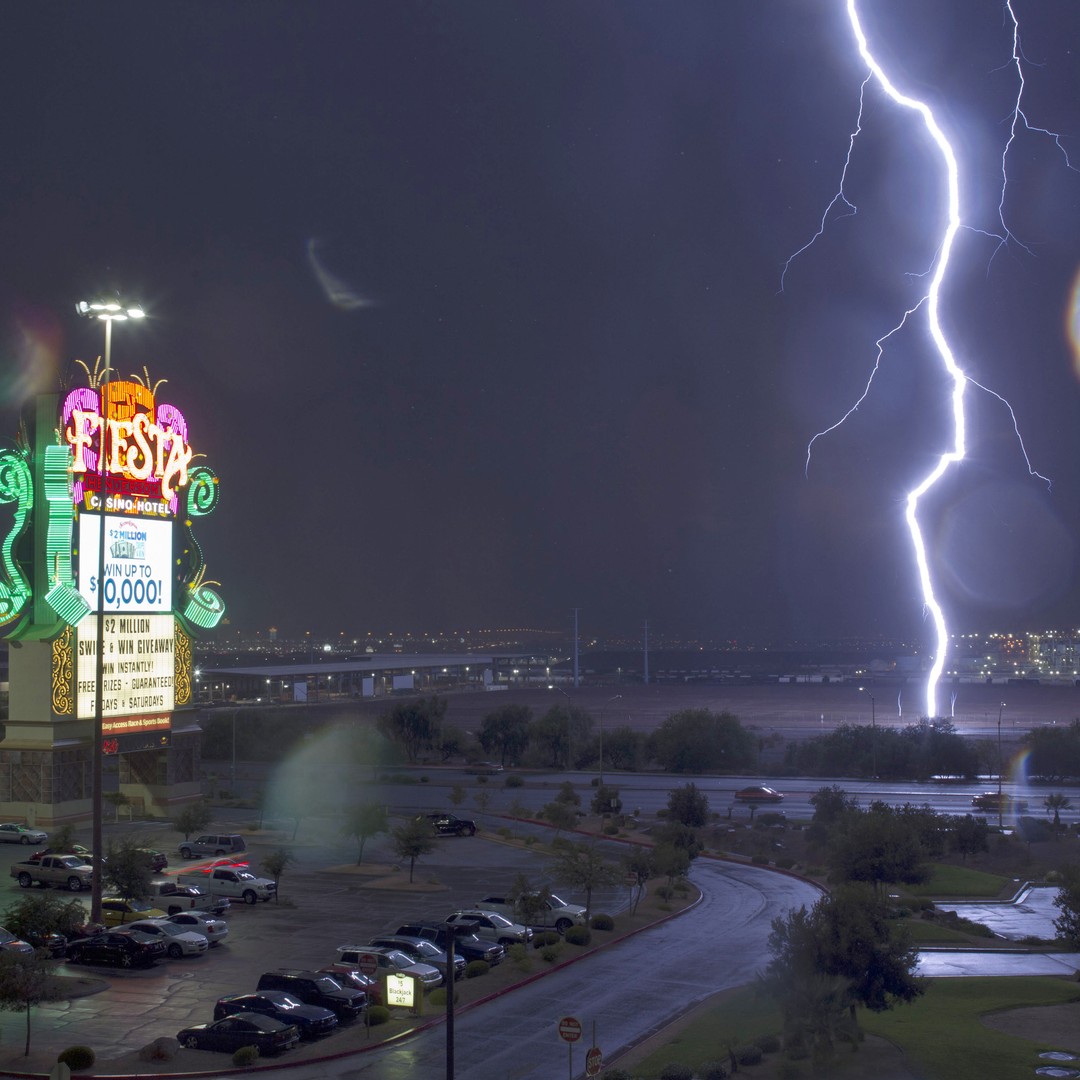The image captures a dramatic nighttime scene where a massive lightning bolt strikes near a Fiesta Casino Motel. The sky is dark and misty, with a significant, jagged lightning bolt emanating from the right, flanked by several smaller branches on either side. The electrical discharge appears to hit a grove of trees around 300 feet from the motel's relatively large, half-full parking lot, enveloped in a mixture of neon lights. The motel's sign, vivid in yellow, orange, pink, and green, highlights offerings such as "Win up to $10,000" and other smaller, less readable text. The scene includes various trees scattered throughout the parking lot and a nearby roadway with signs like "Stop" and "Do Not Enter." The landscape extends further, featuring a highway and hints of a cityscape with residential areas in the distance. The overall ambiance is eerie yet captivating, given the interplay between the ominous weather and the vibrant casino lights.